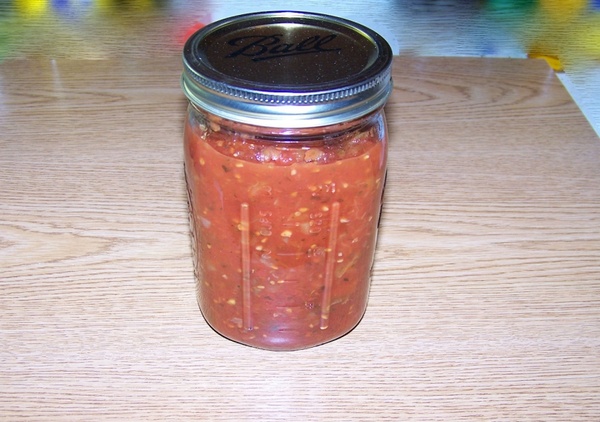This close-up photograph, taken indoors with a flash, features a Ball mason jar filled to the brim with what appears to be homemade salsa. The jar is made of clear glass and showcases the vibrant red salsa, speckled with seeds, pepper flakes, chopped jalapenos, and a tomato puree. The shiny silver lid of the jar prominently displays the "Ball" brand in black cursive. Resting on a light-colored wooden table, likely oak, the image focuses solely on the jar, leaving the background indistinct with faint hints of natural light and blurred colors like yellow and blue at the top. The flash reflects vividly off the metal lid, the glass jar, and the wood grain of the table.